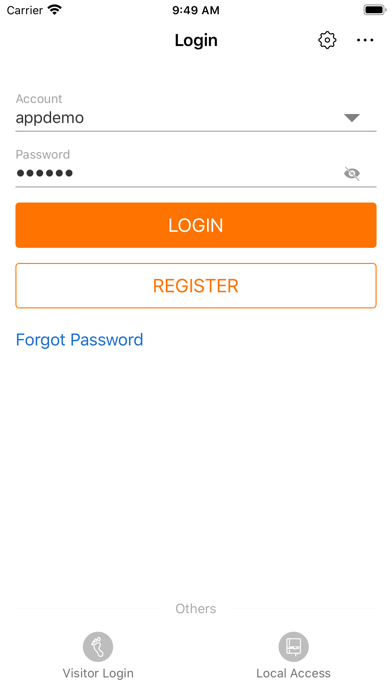In the screenshot depicted, the top-left corner features the 'Cariel' Wi-Fi signal icon, indicating a full 3 out of 3 bars. At the center of the top, the device time reads 9:49 AM. Moving to the top-right corner, the battery icon indicates a full charge. Below the battery icon are the menu and settings buttons.

In the central part of the image, we have several input fields: "Account," "Clean Account," "Name," and "Clean in Password." The account name entered is "appdemon." 

Below these fields are the "Login" and "Register" buttons. Additionally, there is a "Forgot Password" link in blue text.

At the very bottom of the screenshot, there are sections labeled "Others," with two accompanying buttons: "Visitor Login" and "Local Access." The background color of the image is predominantly white.

Thank you for watching.